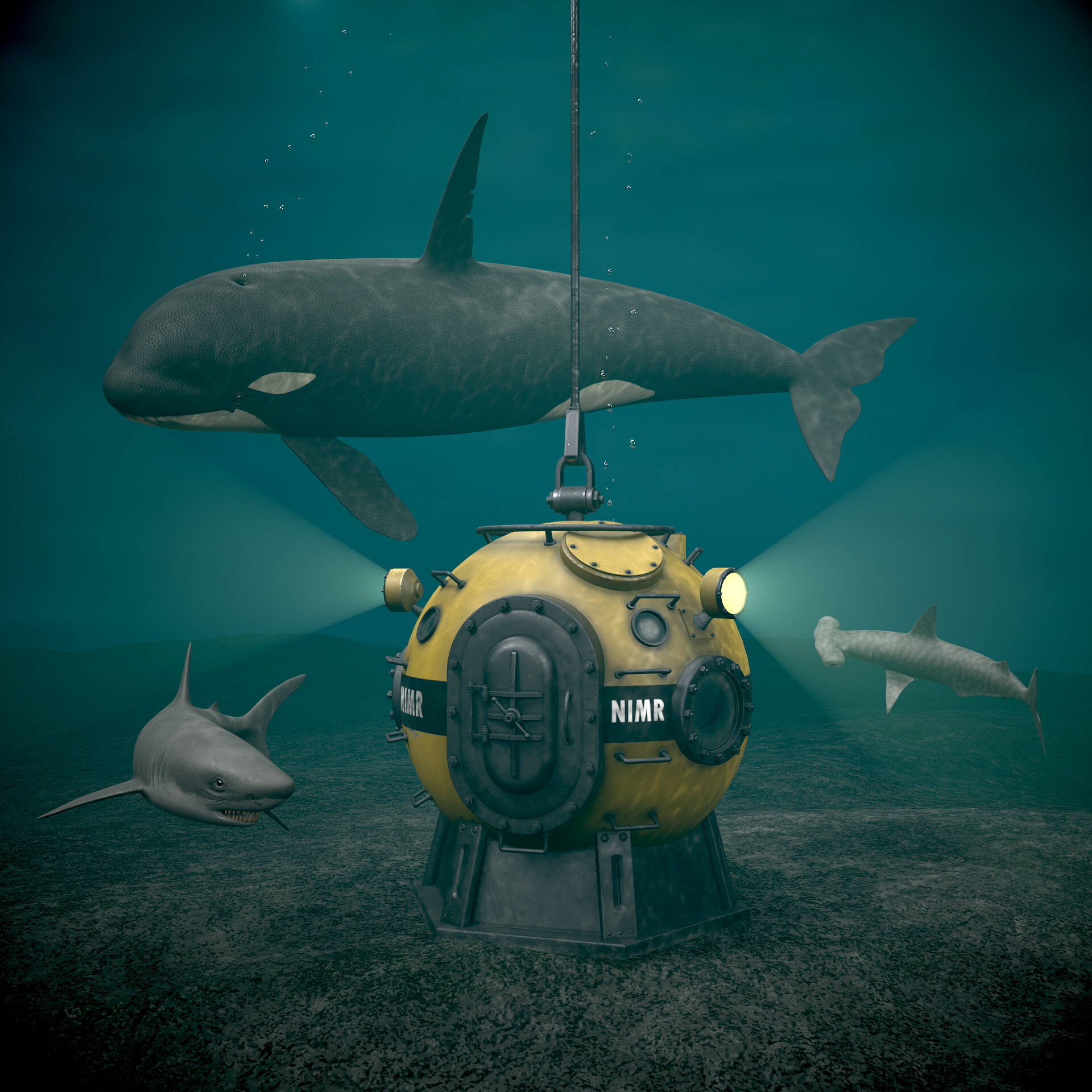The image depicts an underwater scene featuring a computer-generated depiction of an exploration device on the ocean floor. The primary focus is a yellow, round, metallic submersible, often referred to as a baffy spear, equipped with a connecting steel wire at the top, likely for retrieval by a surface ship. Hovering just behind the submersible is an orca, commonly known as a killer whale. To the left of the scene is a shark, potentially a great white, identifiable by a bit of white on its undercarriage. On the right side of the image is another shark, distinguished as a hammerhead by its uniquely shaped head. The overall ambiance of the scene conveys a vivid representation of deep-sea exploration and marine life.